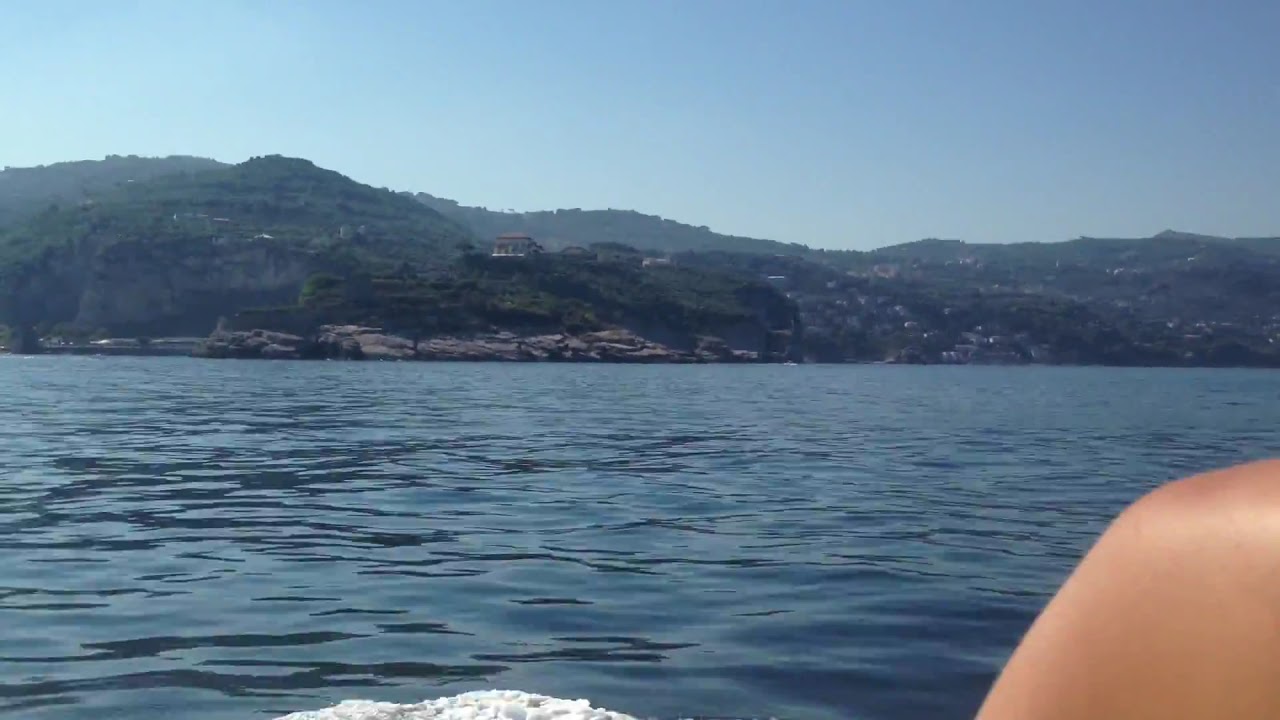The image captures a picturesque coastal scene with a serene and expansive blue ocean dominating the foreground. In the bottom right corner, a person's tanned shoulder and knee indicate their relaxed presence, possibly enjoying the tranquil setting. The coastline features a rocky outcrop with limey, stony formations, leading up to forested, rolling hills of varying heights which are dotted with sparse housing, giving the area a Mediterranean feel. The hills are mostly filled with trees and seem to rise progressively, framing the mid-distance landscape. On the right side, buildings come into view, with one prominent structure near the center, hinting at a less densely populated town rather than a bustling city. Above the tranquil scene is a clear, deep blue sky, with the setting sun suggesting it is late afternoon, around 4pm. This peaceful day at the lake or sea captures the viewer with its natural beauty and calming atmosphere.